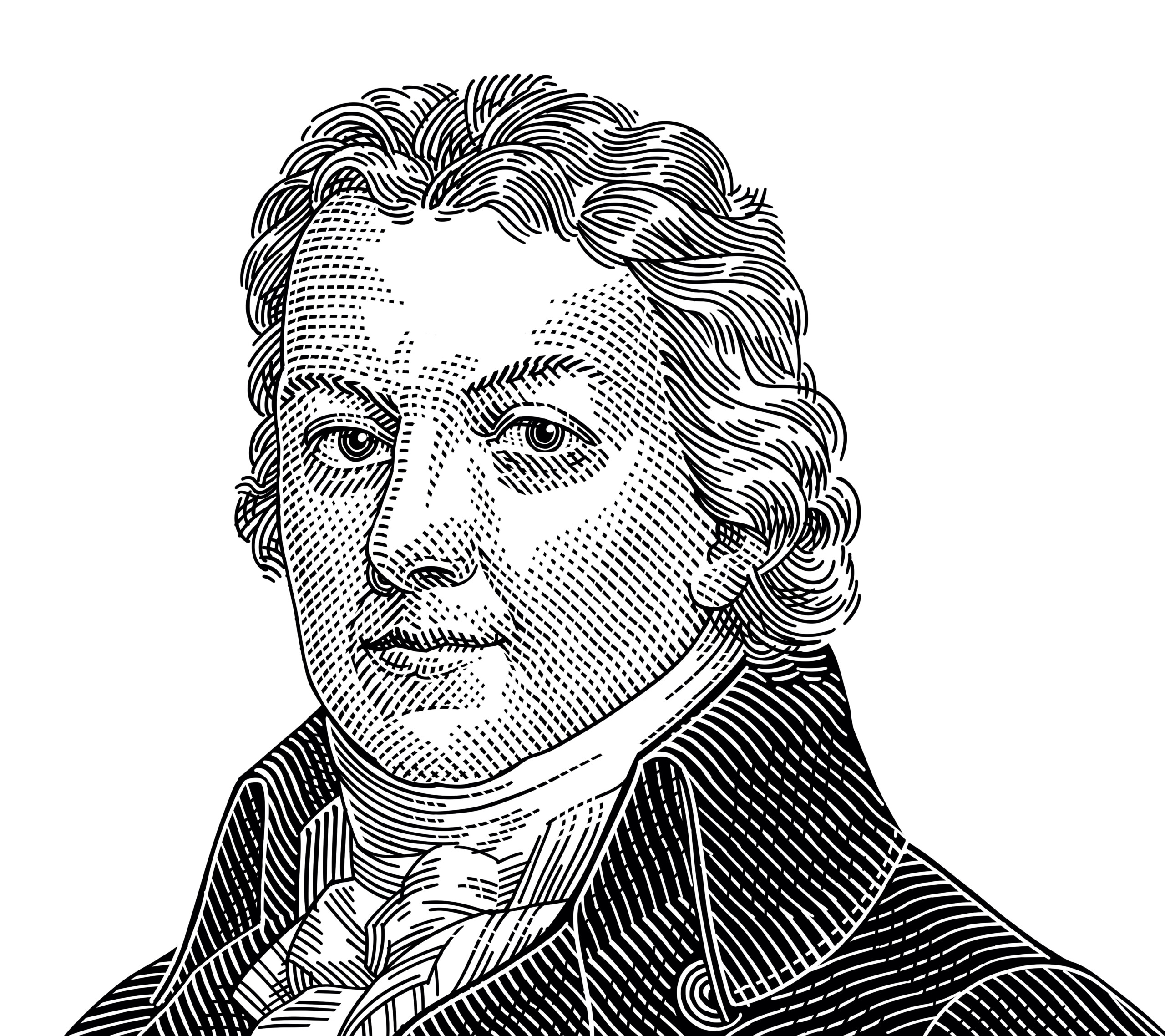This highly detailed black and white pencil drawing is a portrait of Edward Jenner, the 18th-century English doctor renowned for creating the world's first vaccine—against smallpox. The artwork focuses on his head and upper bust, capturing him from the shoulders upwards. Edward Jenner is depicted with short to medium-length curly hair that extends just behind his earlobes, styled in waves that are cleverly illustrated with intricate lines for texture. His eyes are fully open, and the pupils are rendered in black, consistent with the monochrome nature of the drawing.

Jenner is dressed in a distinctive black tuxedo featuring a high collar and an elaborate frilled undershirt that resembles a cravat or scarf around his neck. The fine detailing extends to his jacket, with etched and dashed lines creating texture and shading that accentuate the tuxedo's fabric. A button beneath his collar adds to the clothing detail. His facial features also exhibit meticulous craftsmanship, with dotting and lines illustrating the texture of his skin, including stubble on his cheeks and chin and delicate lines beneath his eyes. His eyebrows are rendered with squiggly lines, adding to the lifelike quality of the portrait. Overall, the meticulous use of lines, dots, and dashes conveys a sense of depth and realism that one might find in historical etchings, reminiscent of the artwork seen on US currency.